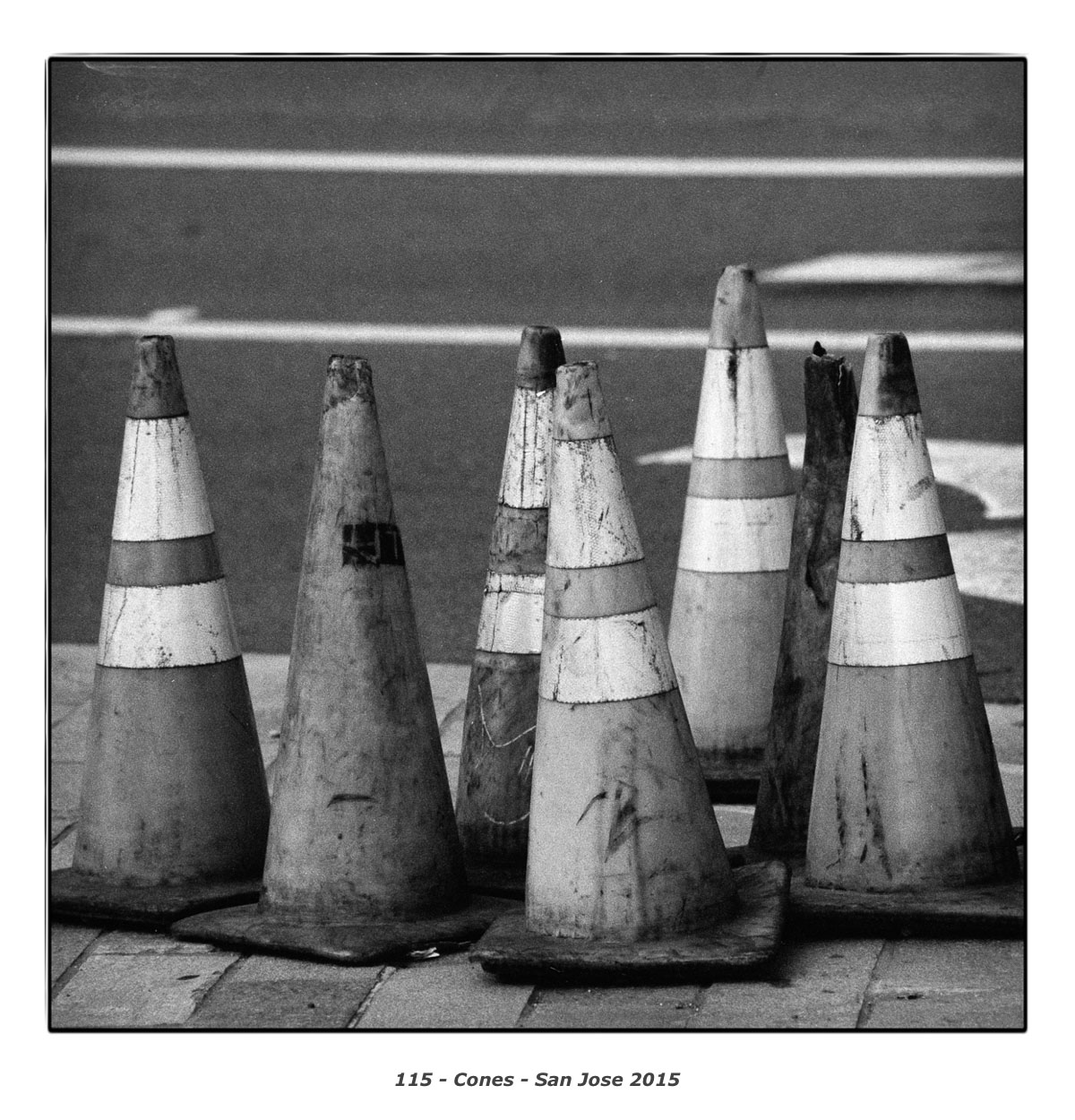This black-and-white portrait-style image prominently features seven battered traffic cones situated on a brick sidewalk. Five of the cones are adorned with double white stripes, while the remaining two cones are solid in color—one noticeably lighter and the other a shade darker. All cones exhibit numerous black markings, indicating significant wear and tear. The background is slightly blurry, revealing a three-lane roadway. At the bottom of the image, a gray font on a white background reads "115-cones-sanjose2015," adding context to this intriguing urban scene.